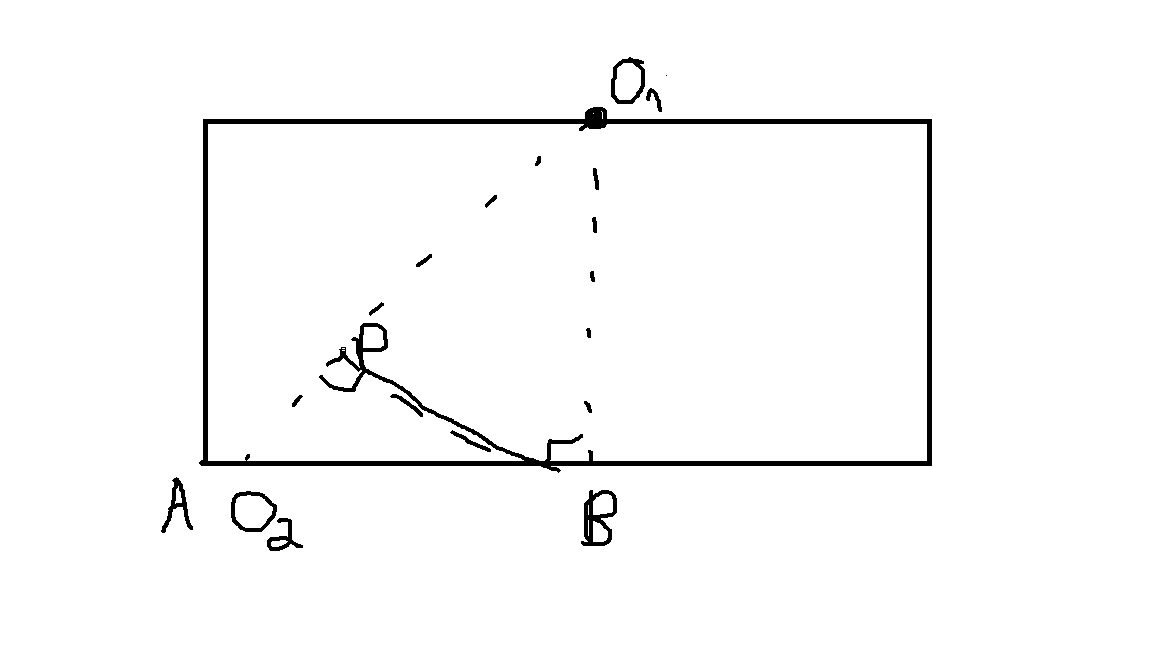In the image, set against a white background, there is a prominent black rectangular outline with a white interior. At the top of the rectangle, the number "0" is positioned next to a small mark. Adjacent to this, there's a large black dot.

From this black dot, a dotted line extends vertically downwards, traversing the entire length of the rectangle. At the bottom of this line, the characters "A" and "O2" are inscribed. On the opposite side of the black dot, at the top, another dotted line descends vertically. Underneath this line at the bottom, the character "B" is noted.

Near the bottom section of the rectangle, but above the inscriptions "A" and "B," there's a diagonal straight line. From this diagonal line, a smaller line ascends, intersecting with the right-side vertical dotted line, resembling two small arms. This smaller line culminates in a flag-like figure near the top. The overall diagram features prominent labels "A," "B," and "0," indicating a structured figure or model with designated points and markers.